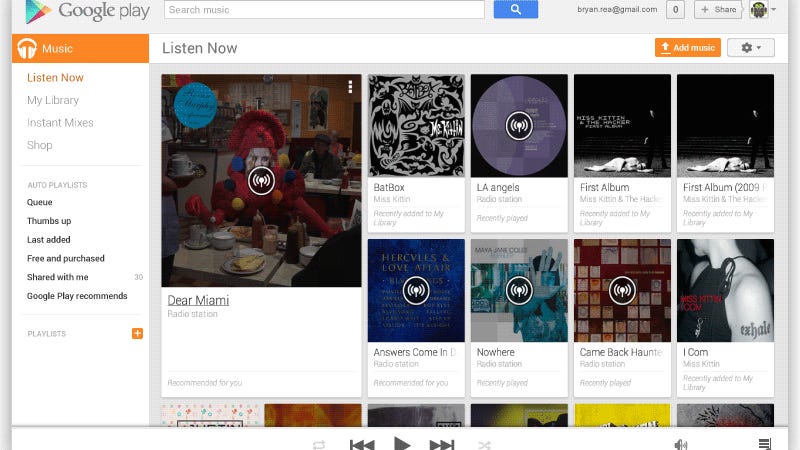This descriptive caption provides a clear and detailed overview of the Google Play webpage, highlighting its layout, navigation options, and main content.

---

The Google Play webpage opens with the Google Play icon on the top left corner, adjacent to a search bar. Displayed prominently next to the search bar is the user’s email, brian.rearay@gmail.com. 

Down the left side of the screen is a vertical navigation menu. This menu includes several options, starting with 'Music', which is currently highlighted. Below 'Music', the 'Listen Now' option is highlighted in orange. Further down, additional options are listed in gray: 'My Library', 'Instant Mixes', and 'Shop'. 

Subsequently, a darker gray section follows, containing more specific subsections: 'Queue', 'Thumbs Up', 'Last Added', 'Free and Purchased', 'Shared With Me', and 'Google Play Recommends'. At the bottom of this vertical menu, there is a 'Playlists' section accompanied by a '+' button, presumably for adding new playlists.

The central area of the webpage is dedicated to the main content, which is titled 'Listen Now' at the top. This section showcases the "Dear Miami" radio station with various songs organized in individual boxes. Among these are 'Bat Box', 'Recently Added to My Library', 'L.A. Angels Radio Station', 'Recently Played', and other entries, offering a comprehensive and organized view of the user’s music and listening options.